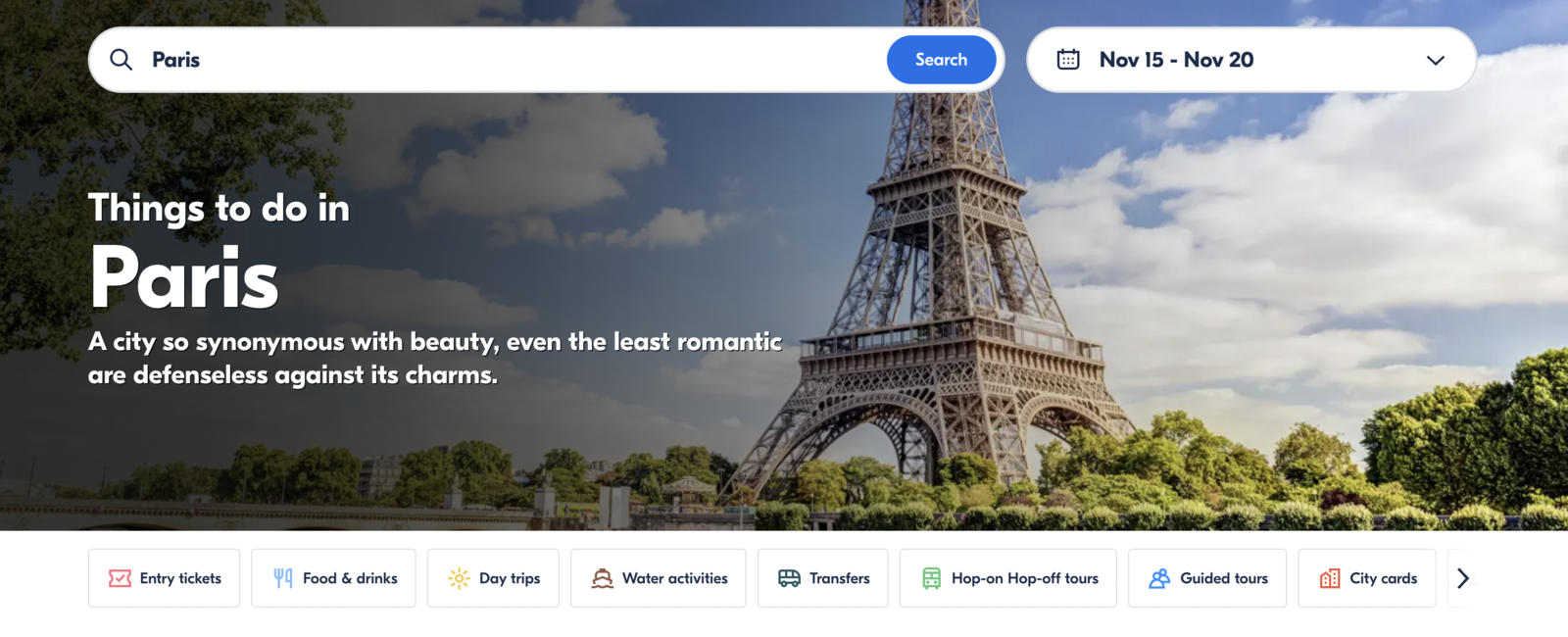### Header Description:

**Explore the Enchanting City of Paris**

The header features a captivating daytime photograph of the Eiffel Tower in Paris, with a stunning play of light and shadow. The left side of the image is slightly darker, gradually transitioning to a brighter, sunlit scene on the right, illustrating the beauty of a sunny day in the city.

In the center of the header is a search box, prominently filled with the word "Paris," indicating a user's quest to discover the city's wonders. Adjacent to it, on the right, is a dropdown box with a calendar icon, displaying the selected dates "November 15th through November 20th."

Text overlay reads: "Things to Do in Paris. A city so synonymous with beauty, even the least romantic are defenseless against its charms."

Beneath the photograph are navigation tabs with corresponding icons, offering diverse activities and services:
- **Entry Tickets** (ticket icon)
- **Food & Drinks** (cutlery icon)
- **Day Trips** (sun icon)
- **Work Activities** (boat icon)
- **Transfers** (bus icon)
- **Hop-on Hop-off Tours** (bus icon)
- **Guided Tours** (user icon)
- **City Cards** (buildings icon)

An arrow icon on the far right suggests further navigation options.